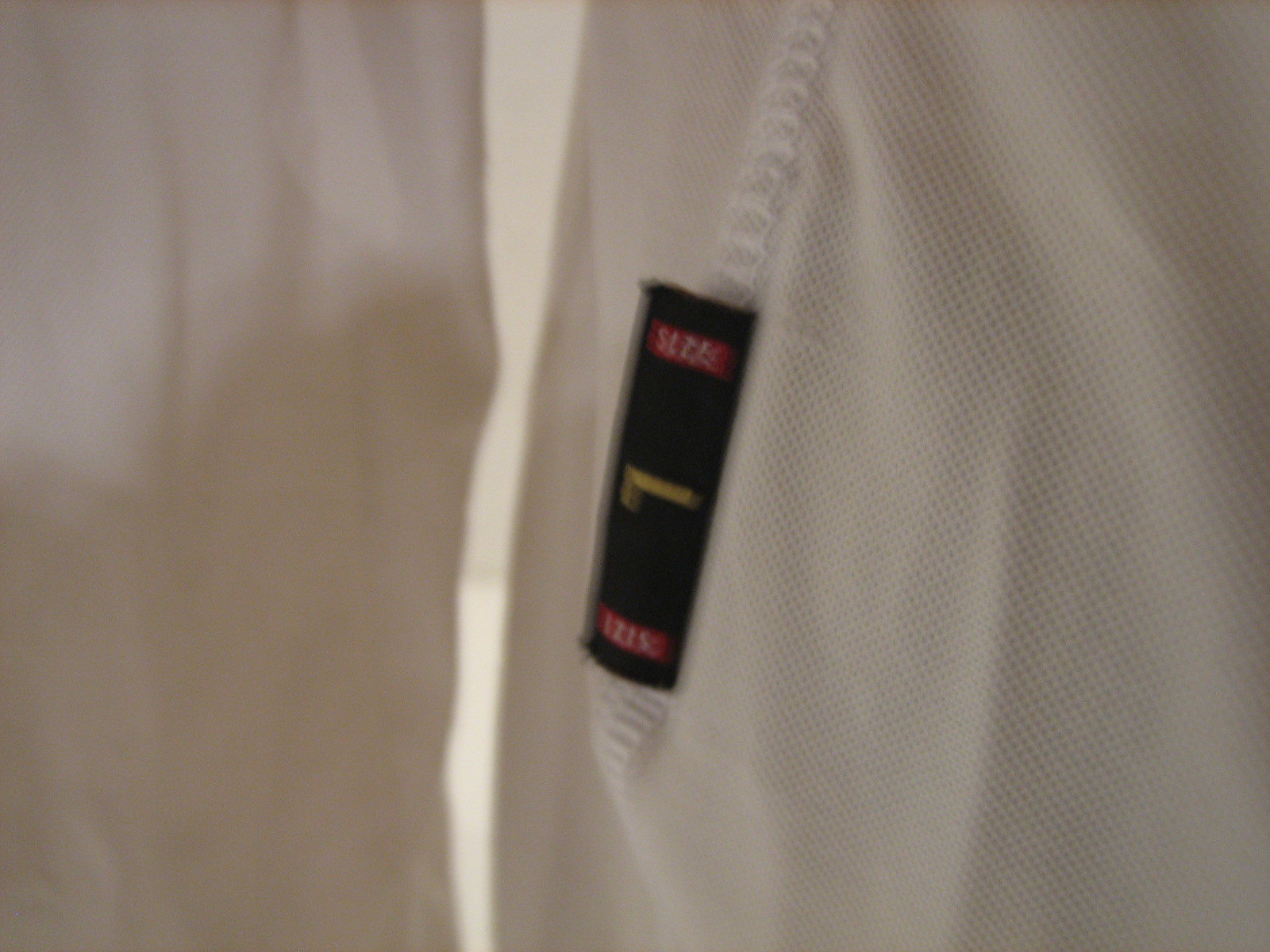In this image, a blurred white garment can be seen, featuring a subtle waffle texture on its fabric. The item appears to be a polo shirt, with a prominent fold running vertically down the center. Just to the right of this fold, a seam is visible. A black label is present on the garment, adorned with red bars at both the top and bottom. The label has white lettering, which seems to spell out "S-L-Z-A" or a similar combination of letters. Additionally, there is a yellow design to the left of the label, consisting of a square and an attached rectangle extending horizontally to the right.